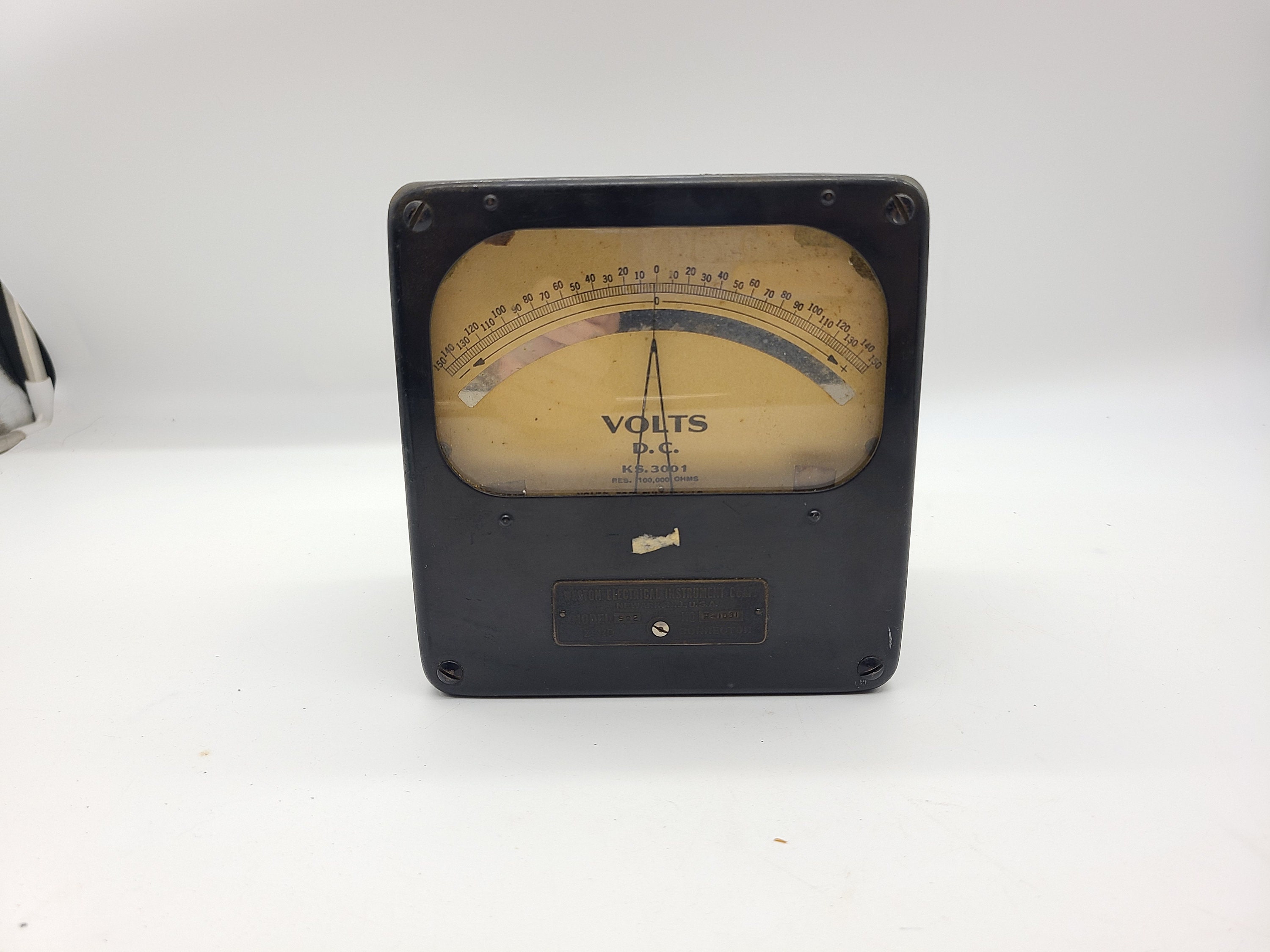The image displays a piece of vintage electrical measuring equipment, likely a voltmeter, set against a white background. The instrument is enclosed in a squarish black case with rounded corners and features a flathead screw in each corner. Centrally positioned on the device is a rectangular window with rounded edges, displaying an arched scale marked with numbers ranging from 0 to 150 in both directions. Below this arched scale, the text "VOLTS DC" is clearly visible. The scale includes a pointer indicating measurements and a small mirror beneath it, assisting in reading accuracy. There is an additional marking, "KS3001," on the device. On the left side of the image, a partially visible black and white object can be seen, potentially the base of a pole, adding to the image’s intricate details. The overall appearance suggests the instrument is quite old, especially given the yellowed and worn look around the numerical display.